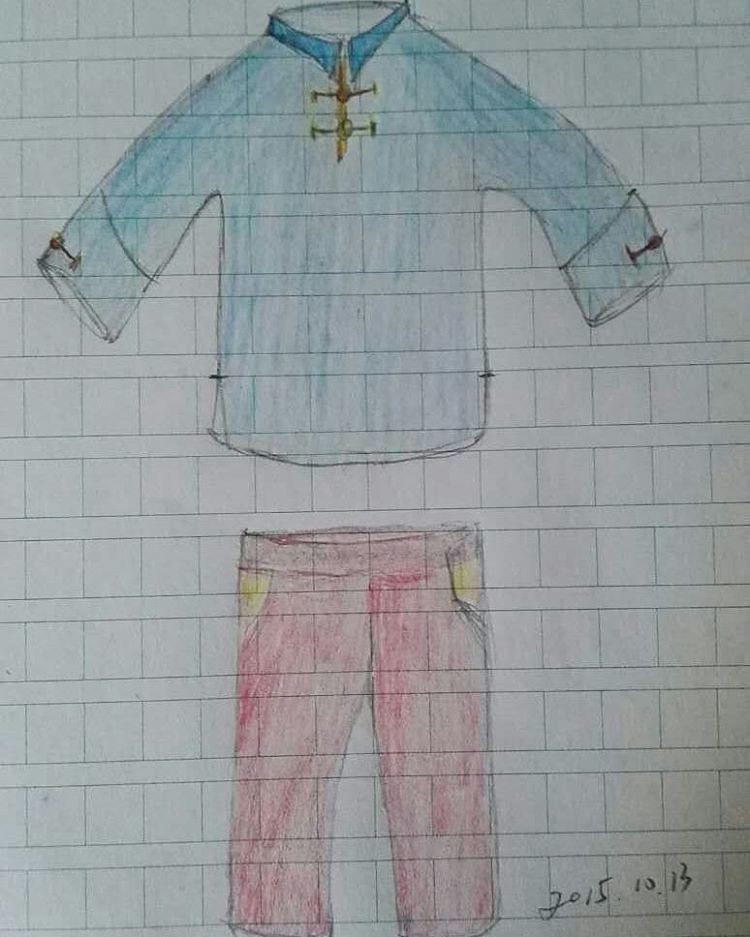This image features a detailed pencil and colored pencil drawing on graph paper, with a grid of squares forming the backdrop. At the top of the drawing is a shirt rendered in shades of blue, complete with two small button ties at the neck and a dark blue collar. The sleeves of the shirt also feature the same button tie detail. Below the shirt, there is a noticeable gap before the artist depicted a pair of red pants. These pants are highlighted by distinctive yellow pockets. In the bottom right corner of the page, the artist has inscribed the date "2015.10.13" in black ink.